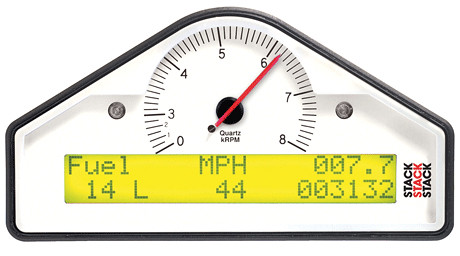This image showcases a tachometer with a predominantly white background. The tachometer has black numerals and markings, while the needle, used to indicate readings, is red and positioned on a central black pivot point. Surrounding the tachometer's white face is a black border, creating a distinct frame. On either side of the tachometer, small indicator lights, potentially for turn signals, are visible.

Beneath the tachometer, there is a yellow digital display panel providing various readings:
- Fuel level: 14 liters
- Speed: 44 (units not specified, likely km/h or mph)
- Additional metrics: 007.7 and 003132 (exact meaning unclear)
- Tachometer reading: 6.2 (units not specified, likely thousand RPM)

There is also repetitive text that says "stack, stack, stack" in black letters. The precise context of these numbers is ambiguous but may relate to the vehicle's performance data rather than the tachometer itself.